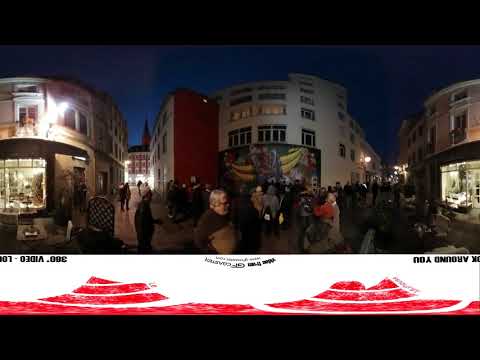This horizontal rectangular image appears to capture a nighttime scene in a small, European-style city square. The top portion of the image likely depicts a lobby or storefront, with noticeable glass doorways on the left side and what could either be a television screen or another room entrance on the right. The center of the image is dimly lit, emphasizing the dark tonal quality of the overall scene.

In the middle section of the image, a gathering of people is visible, suggesting a social or touristic atmosphere, possibly around outdoor restaurant tables. People are milling around narrow streets, which give the impression of leading to or from significant buildings, one of which includes a tower. A prominent figure in the center—a man with gray hair, glasses, a beard, and wearing a sweater—draws particular attention. 

Dominating the lower portion of the image is a dark black band featuring red curved abstract designs interspersed with white lines. Within this band, there is upside-down text reading "300 video," "GF company," and "look around you," which adds an additional element of curiosity to the composition. Overall, the juxtaposition of architectural detail, human activity, and graphic design creates a richly layered and atmospheric portrayal of a city square at night.